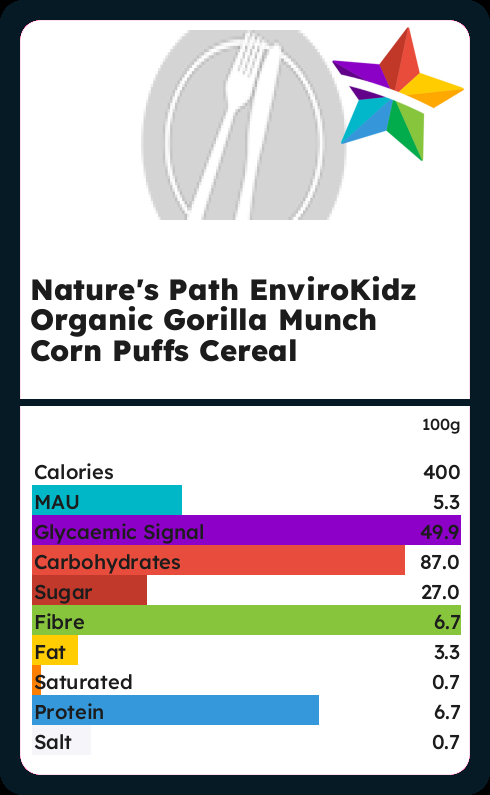In the image, we see a detailed view of a cereal box and its nutritional information. At the top, the product is identified as Nature's Path EnviroKids Organic Gorilla Munch Corn Puffs Cereal. The box prominently displays the name "Gorilla Munch Corn Puffs" in bold green lettering. The front of the box features an engaging illustration of a gorilla, along with an appetizing image of a bowl filled with corn puffs and milk being poured into it.

Below the image of the cereal box, a table lists detailed nutritional values: 

- Calories: 400
- MAU: 5.3
- Glycemic Signal: 49.9
- Carbohydrates: 87.0g
- Sugar: 27.0g
- Fiber: 6.7g
- Fat: 3.3g
- Saturated Fat: 0.7g
- Protein: 6.7g
- Salt: 0.7g

Additionally, there is a "calorie star" symbol at the bottom. In the left-hand corner, there is a row of seven small boxes, though their exact purpose or meaning isn't clear.